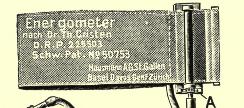In the photograph, there is a prominently displayed light yellow sign. At the center of this sign, a large black rectangular area resembling a billboard is illustrated. The text on this black area reads: "Energometer, NAC Dr. T.H. Kristin D.R.P. 225503 SCHW.PAT.NUM50753." Below this text, there is additional smaller text, which is not legible. On the bottom right corner of the black area, a distinct black letter "A" is visible. It appears that the sign could be related to a patent or a scientific instrument, given the technical nature of the information provided. Additionally, there is an indeterminate object protruding from the bottom left side of the sign, though it is not clearly identifiable in the image.